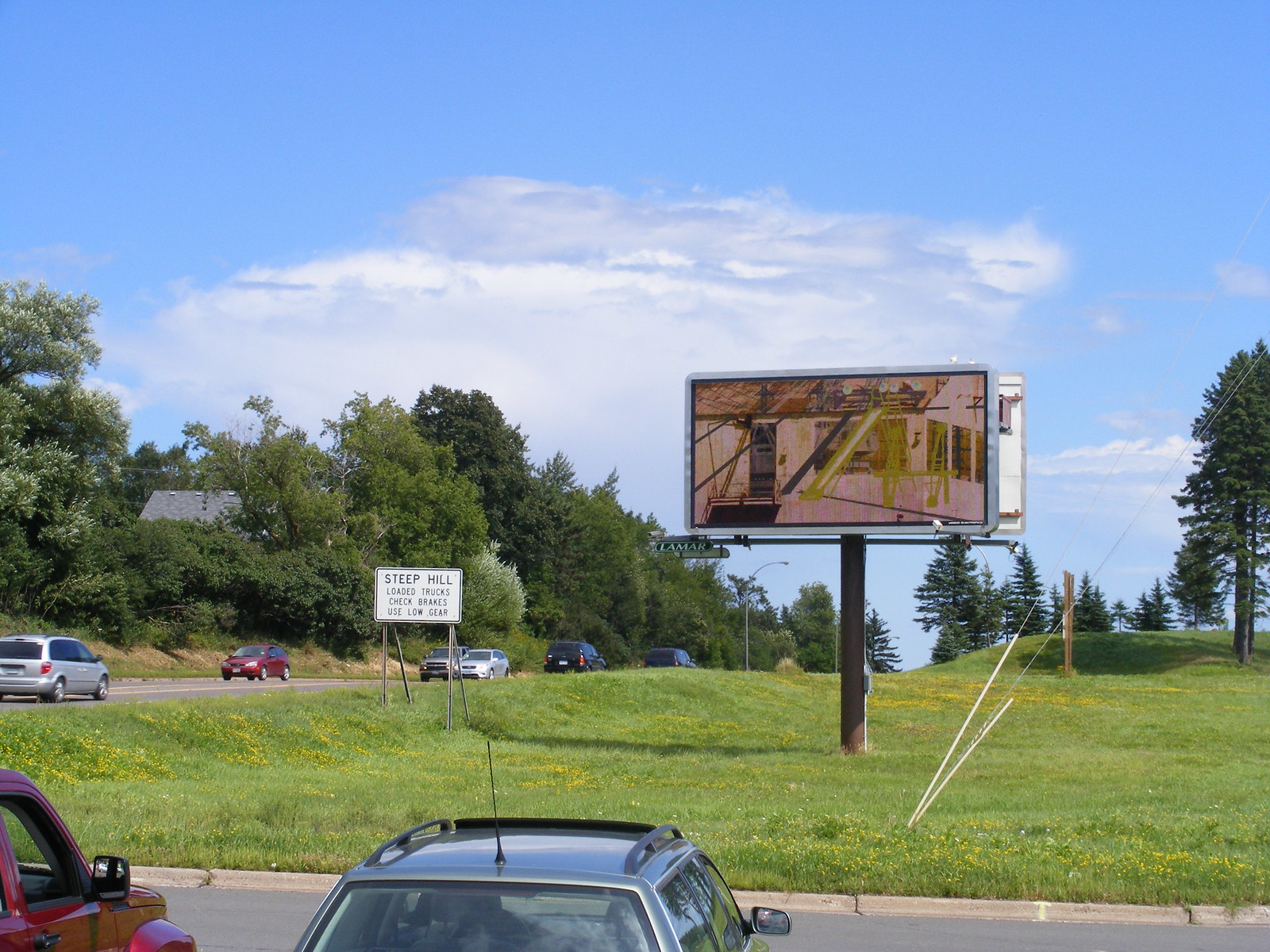This photograph captures a vivid outdoor scene in a sunlit afternoon, depicting a diverse mix of elements blending naturally. Standing prominently in a field of bright green grass dotted with yellow flowers, a high-mounted digital billboard displays an image of a house under construction, with framed walls and a foundational roof. Adjacent to the billboard, a white signboard reads, "Steep Hill, Loaded Trucks, Check Brakes, Use Low Gear."

The parking lot in the foreground features a red vehicle in the bottom left corner and a station wagon with a roof rack and antenna almost centered at the bottom edge. To the left, a road, bordered by the green verge, has traffic flowing in both directions. This road leads towards the middle of the image, where beyond the road, lush trees in different shades of green, including one with white flowers and a set of fir trees on the right side, provide a picturesque backdrop. Among these trees on a hill, the roof of a house peeks out. The sky overhead is a brilliant blue, transitioning to pale grey and white fluffy clouds near the horizon, adding a touch of tranquility to the bustling scene below.